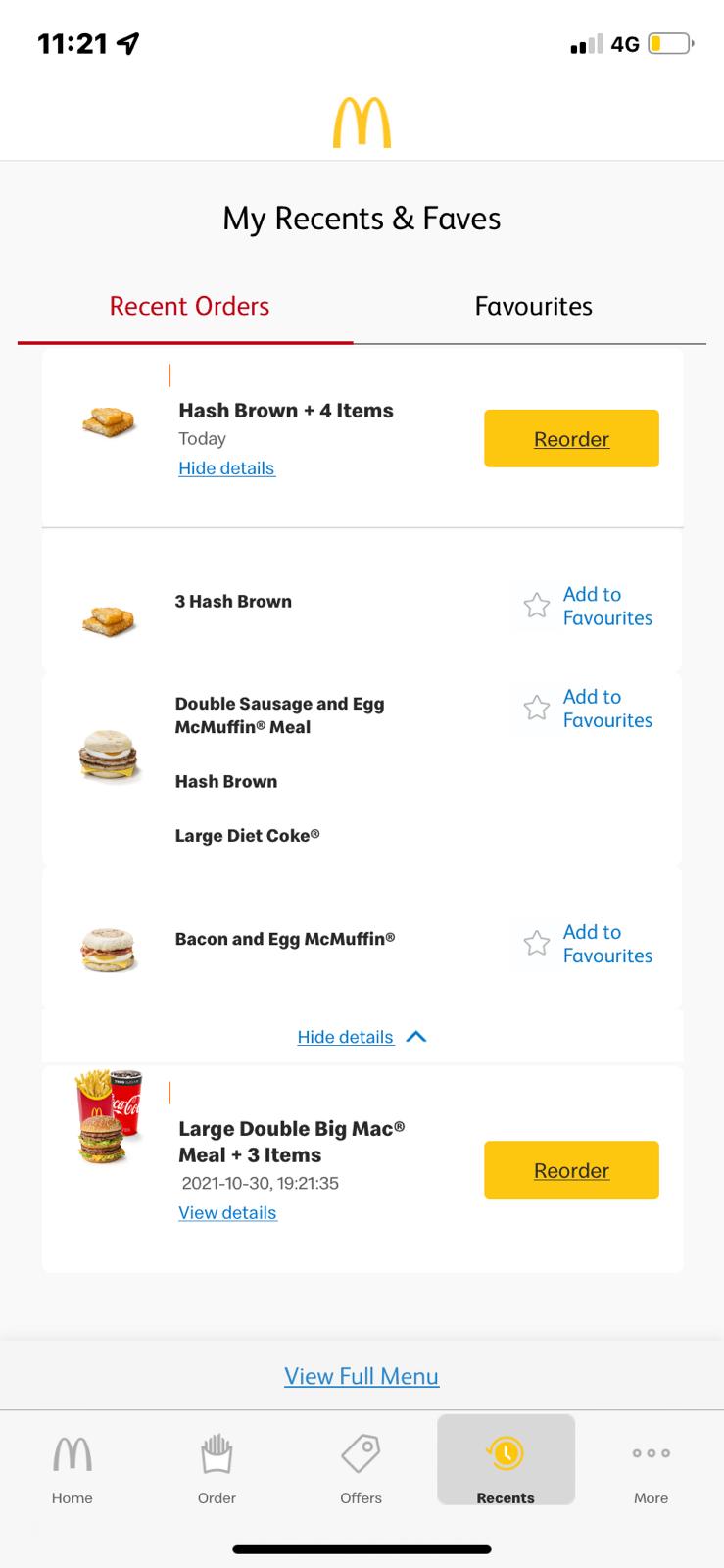The screenshot displays the home screen of a mobile application at 11:21 AM, as indicated by the time at the top of the screen. The phone shows a signal strength of 2 out of 4 bars, with a nearly depleted battery. Dominating the center of the screen is the McDonald's logo, situated above a grey box labeled "My Recent and Faves."

The grey box is divided into two tabs: "Recent Orders" on the left, which is highlighted in purple, and "Favorites" on the right. Below this section, the screen transitions to a white background displaying recent orders. The first entry lists "Hash Brown plus 4 items today," followed by a blue hyperlink labeled "High Detail" and a yellow "Reorder" button.

Further information reveals the items included in the order: 3 Hash Browns, a Double Sausage and Egg McMuffin Meal, Hash Browns, a Large Diet Coke, and a Bacon Egg McMuffin. Each item has an adjacent blue hyperlink with the option to "Add to Favorites."

The subsequent section details another order: "Large Double Big Mac Meal plus 3 items," with a timestamp of "2021-10-30 19:21:35." Additional options include a blue hyperlink for "View details" and a yellow "Reorder" button on the right.